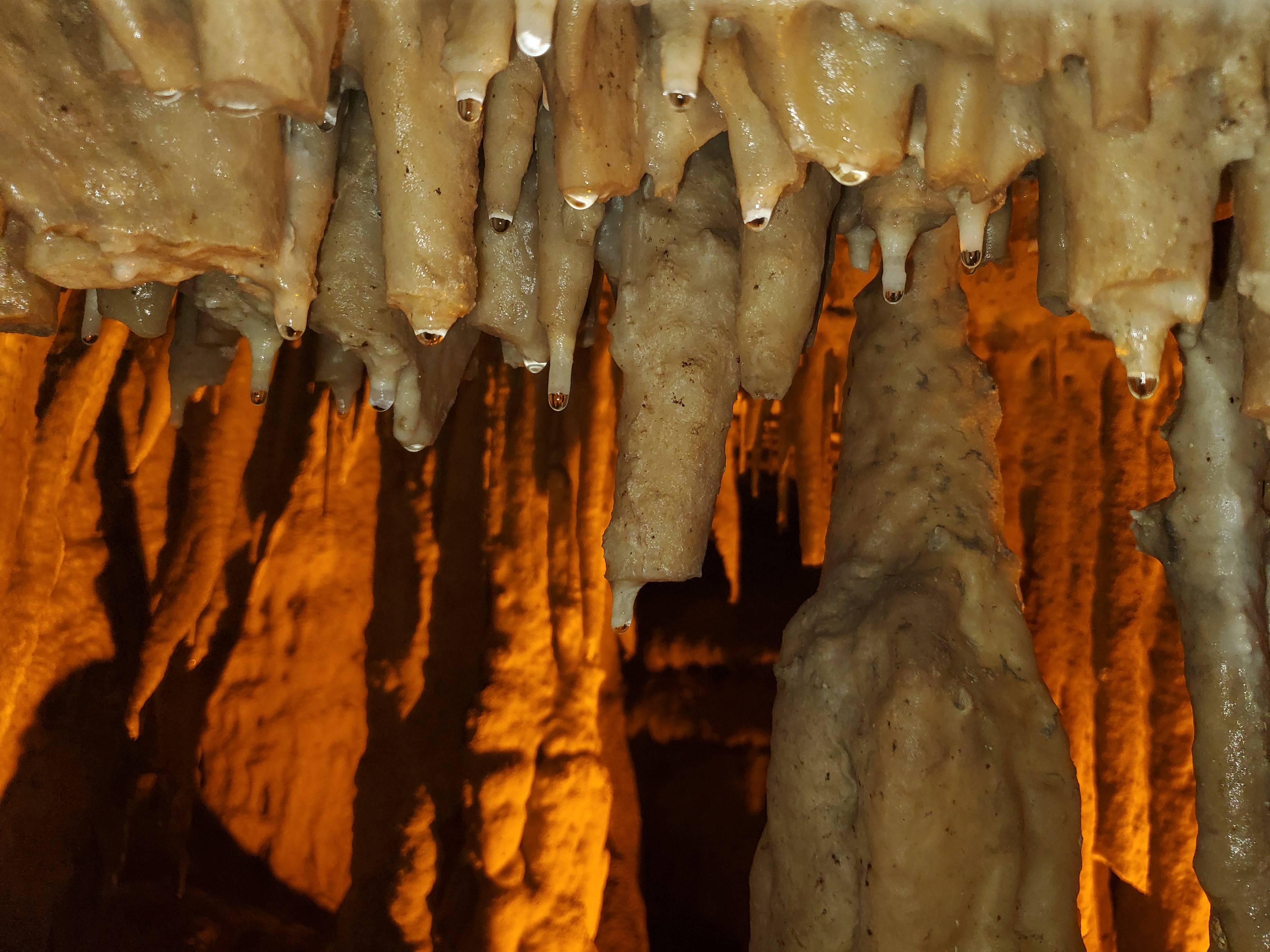Inside the illuminated depths of a cave, a mesmerizing scene unfolds. An unseen orange fire casts a warm glow, highlighting the moist, tan-gray speleothems that adorn the interior. Dominating the center are two imposing stalagmites, their wet, almost glassy surfaces stretching upward towards a ceiling adorned with a variety of low-hanging, tentacle-shaped stalactites. Water continuously drips from the stalactites, pooling at their tips and down their lengths, contributing to their shiny, almost rubbery appearance. The stalactites, varying in size and shape from thick, flat-tipped formations to slender, pointy ones, create a dynamic display that contrasts with the dark recesses of the cave's backdrop. On the bottom right, the firelight creates a gradient of bright yellow to darkness, accentuating the cave's natural, bone-colored stone textures. The overall ambiance is one of eerie yet captivating natural beauty, where rock structures potentially mimic organic forms, blending seamlessly into the cavernous landscape.